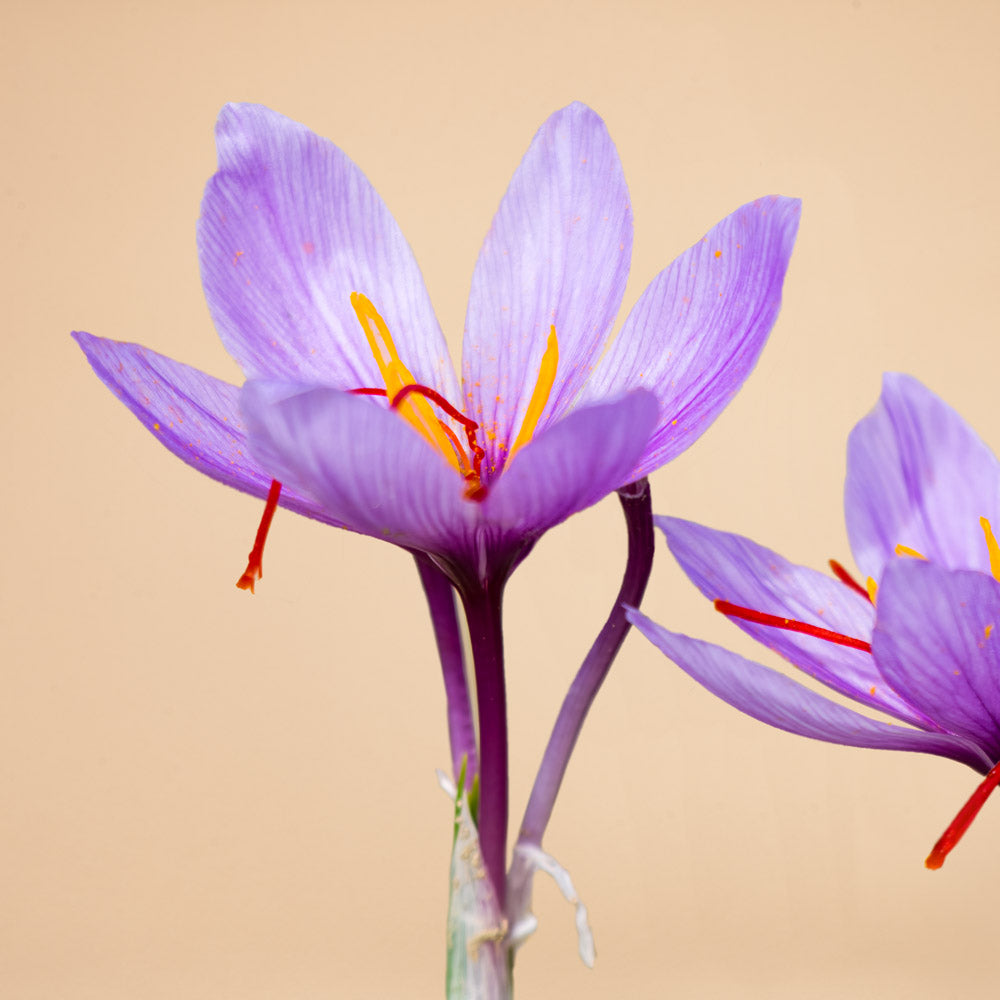In front of a light brown, peachy-beige background, the photograph showcases a striking lavender crocus flower, with its delicate lighter interior and darker outer petals. Prominently in the center, the crocus displays vivid yellow stamens and distinctive red prongs that hang over the edges. The stem of the flower, which is purple and green, rises from green leaves at the bottom of the image. A second flower leans in from the right side of the picture, partially visible, with four visible petals and similarly colored red and yellow elements in the center. The background is solid and unadorned, drawing focus entirely to the vivid floral subjects.